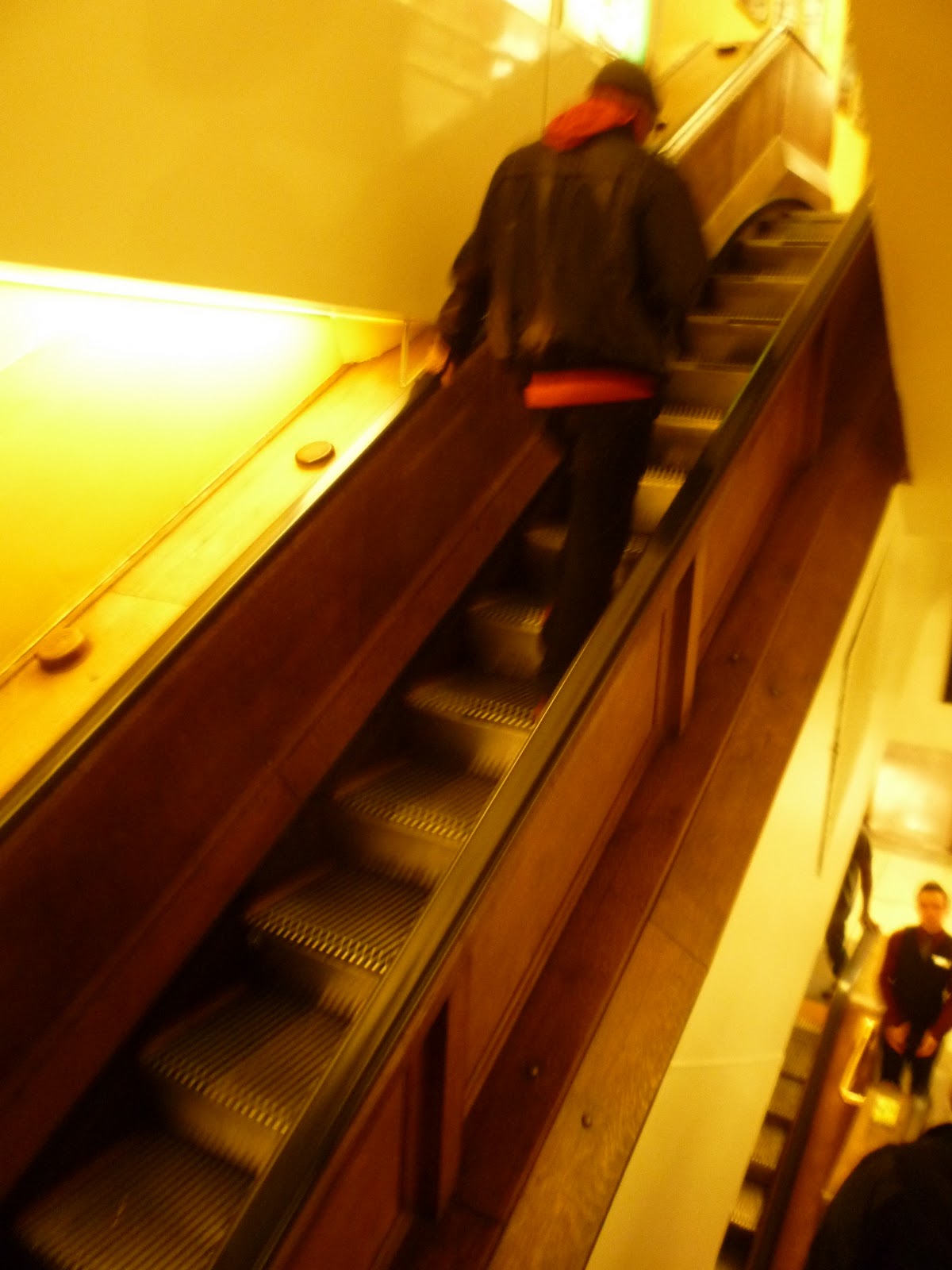In this blurry and washed-out photograph, captured with a yellow tone, a man on an escalator dominates the scene. The escalator runs diagonally from the bottom left to the top right. The man is centrally placed in the upper half of the image, wearing a red hoodie underneath a black jacket, paired with black pants. His left hand grips the left rail of the escalator, and his head is bowed slightly as he appears to look towards his hand. The man wears a black cap, adding to his noticeable attire amidst the predominantly yellow and brown hues. The steps of the escalator exhibit a gunmetal color, further enveloped by the warm yellow lighting. In the blurred background, at the bottom right corner, another man stands under and behind the escalator, his actions and purpose unclear. The overall warmth of the image restricts the palette, highlighting blacks and browns more distinctly. The setting appears to be an underground or subway environment, contributing to the photo's uniquely hazy and sepia-like quality.